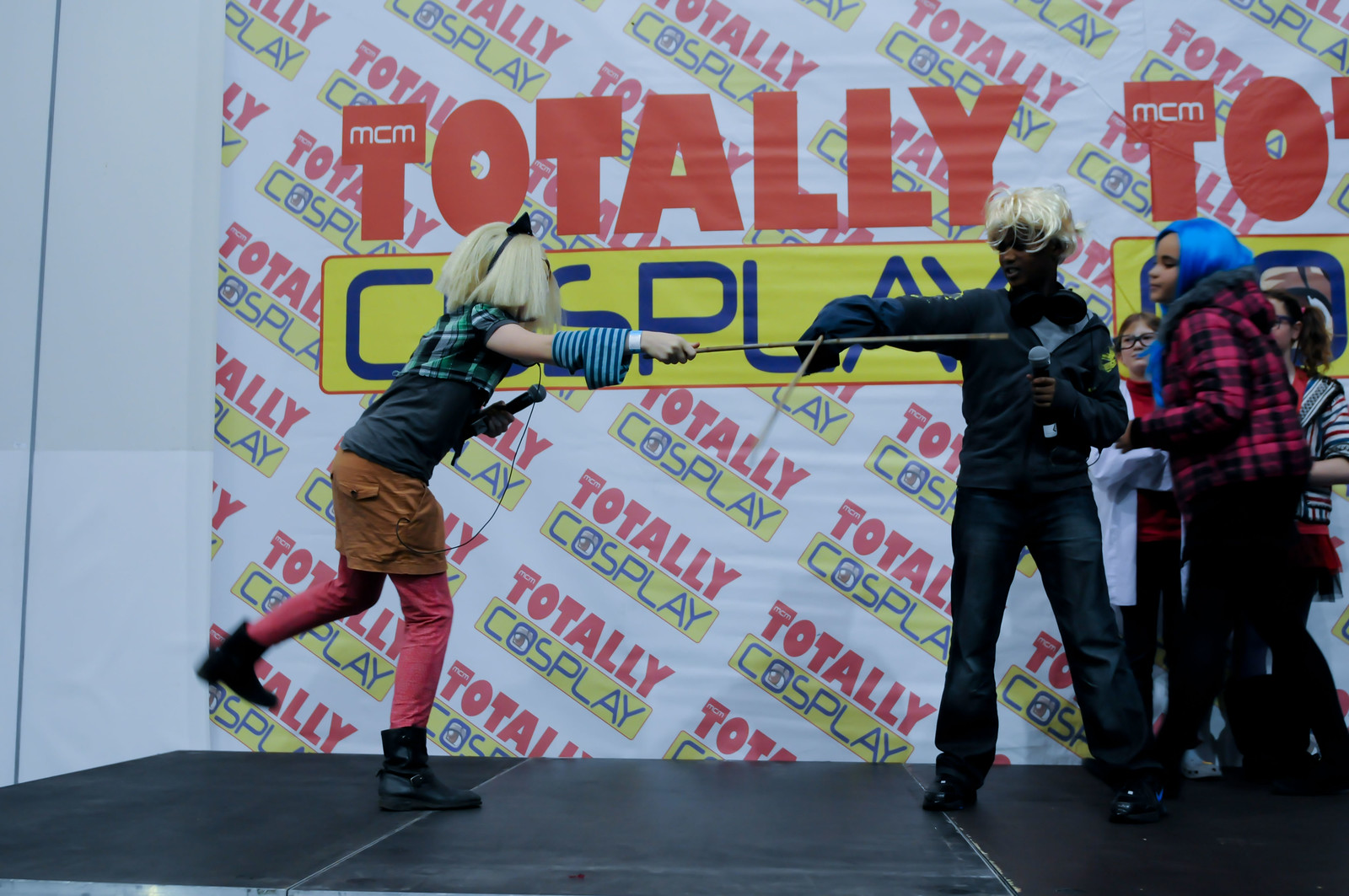The photograph captures a scene from a cosplay convention on a black stage, with a white wallpaper backdrop repeatedly printed with the words "MCM Totally Cosplay." On the left side of the stage, a woman with platinum blonde hair adorned with a red bow is dressed in a checkered green and black shirt, brown shorts with pants underneath, and black boots. She is holding a yardstick-like metal stick pointed to the right and a microphone as she stretches out. To the right of her stands another person wearing a black top and dark blue jeans with brown hair, also holding a microphone. Additionally, there is a black woman with a separate stick angled perpendicularly, seemingly interacting with the blonde woman’s stick. Further to the right, a girl with blue hair looks on as the scene unfolds.